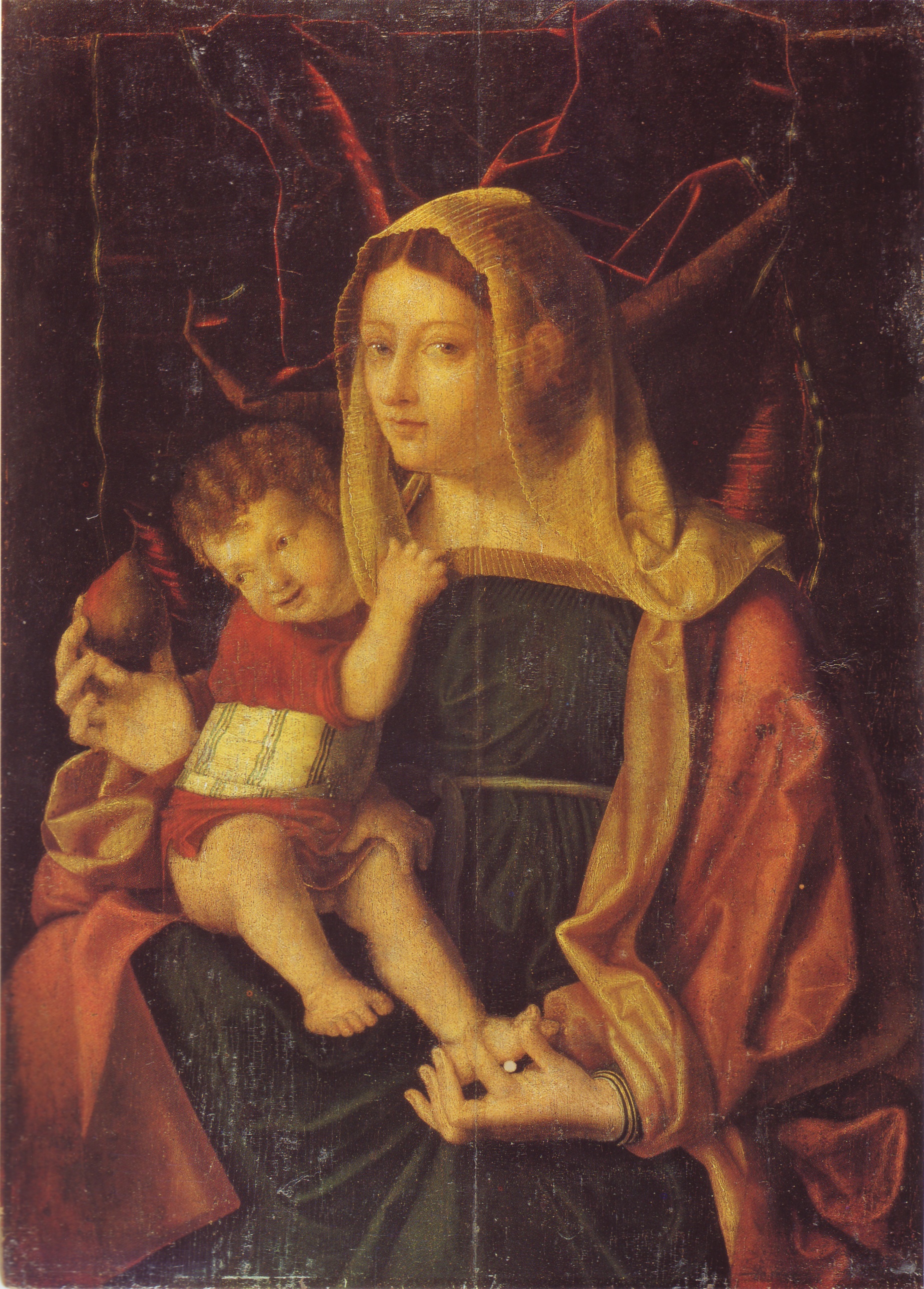This painting depicts a mother and her child in a finely detailed Renaissance era style. The mother, a fair-skinned Caucasian woman with brown hair, is looking directly at the viewer with captivating eyes. She is adorned in a traditional dark green dress accented with gold that graces her chest, and she wears a red shawl draped over her shoulders. Her head is covered with a transparent, yellowish headscarf that still allows her ear to be visible beneath it.

Seated, she cradles her child, a young boy with short, orangish-brown hair, on her lap. The child, dressed in a red top featuring a black and white band around the waist, is gazing intently at a piece of fruit—a pear or fig—that the mother holds close to his face with her right hand. Her left hand tenderly supports the boy's foot, creating a tender interaction between them.

The background is a rich, velvety red material, elegantly crumpled, adding depth and an intimate atmosphere to the composition. The texture and color of the background suggest an element of luxurious warmth, characteristic of the painting's old-world charm.